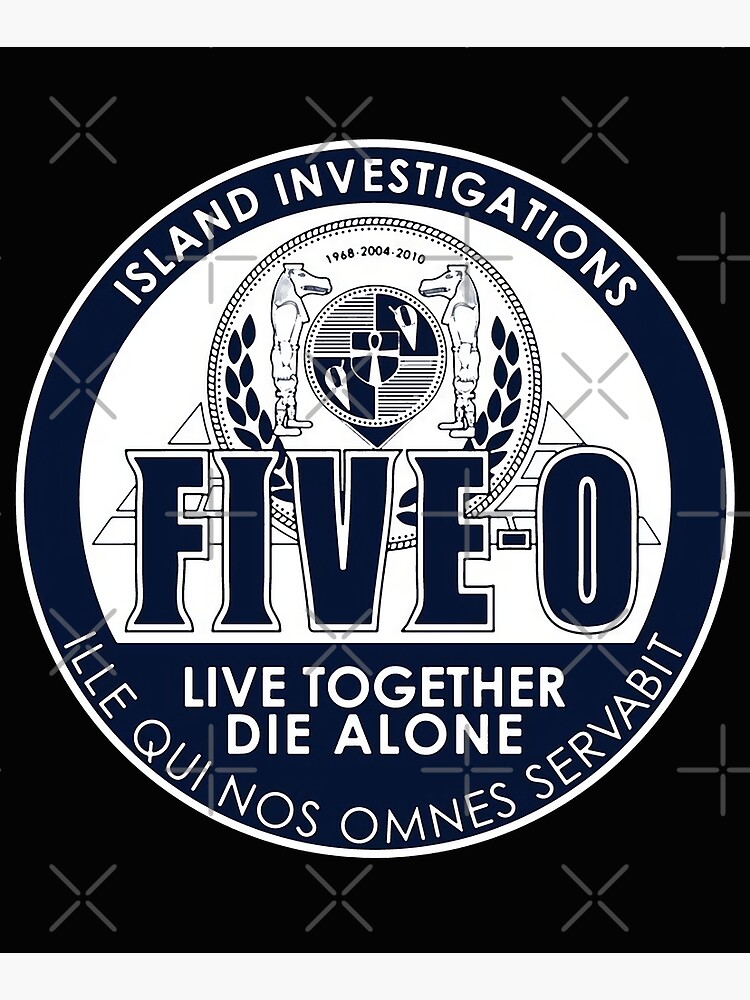The image depicts a logo set against a dark blue background with a white border. At the top, in white lettering, it reads "Island Investigations." Encircling the bottom, it reads "ILLE QUI NOS OMNES SERVABIT" in white letters. The center of the logo features a detailed seal: two figures with human bodies and hippo heads, reminiscent of Egyptian gods, face each other. Between them, there's a smaller circle containing an ankh. Below this seal, large dark blue letters spell out "5-0" and beneath that, in white letters, is the phrase "Live together, die alone." The image appears to be on a black backing with X's and pluses, indicating a non-replicable, copyright-protected photograph.